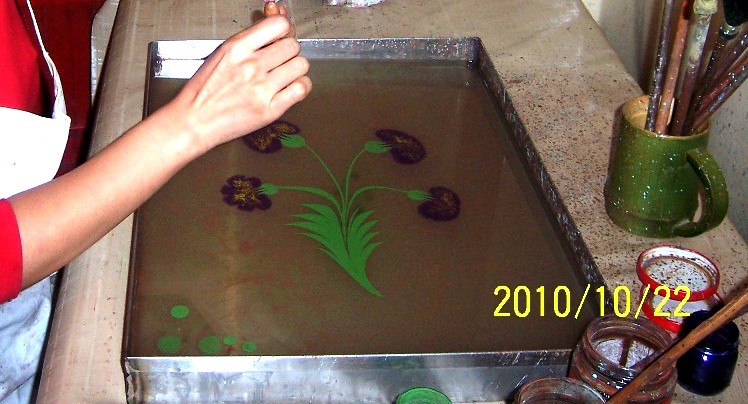This photograph captures a detailed scene of an individual engaged in silk screening artwork on a floral design inside a large, silver, metal cookie sheet. The deep stainless steel pan rests securely atop a tiled countertop. The focal point of the image is the intricate floral design, showcasing four purple flowers with yellow splotches that intensify towards the centers, branching out from four stems and complemented by a large leaf at the base.

The artist's workspace is organized, featuring a green coffee cup housing paint brushes and open jars of paint situated in the bottom right corner of the frame. Indicating a dynamic process, the individual is seen standing to the left of the countertop, extending an arm over the tray, seemingly pouring a liquid solution or possibly working with a plastic resin to complete the vibrant flower image. The scene is bustling with creativity, with the presence of the tools and materials hinting at a meticulous and engrossing artistic endeavor.